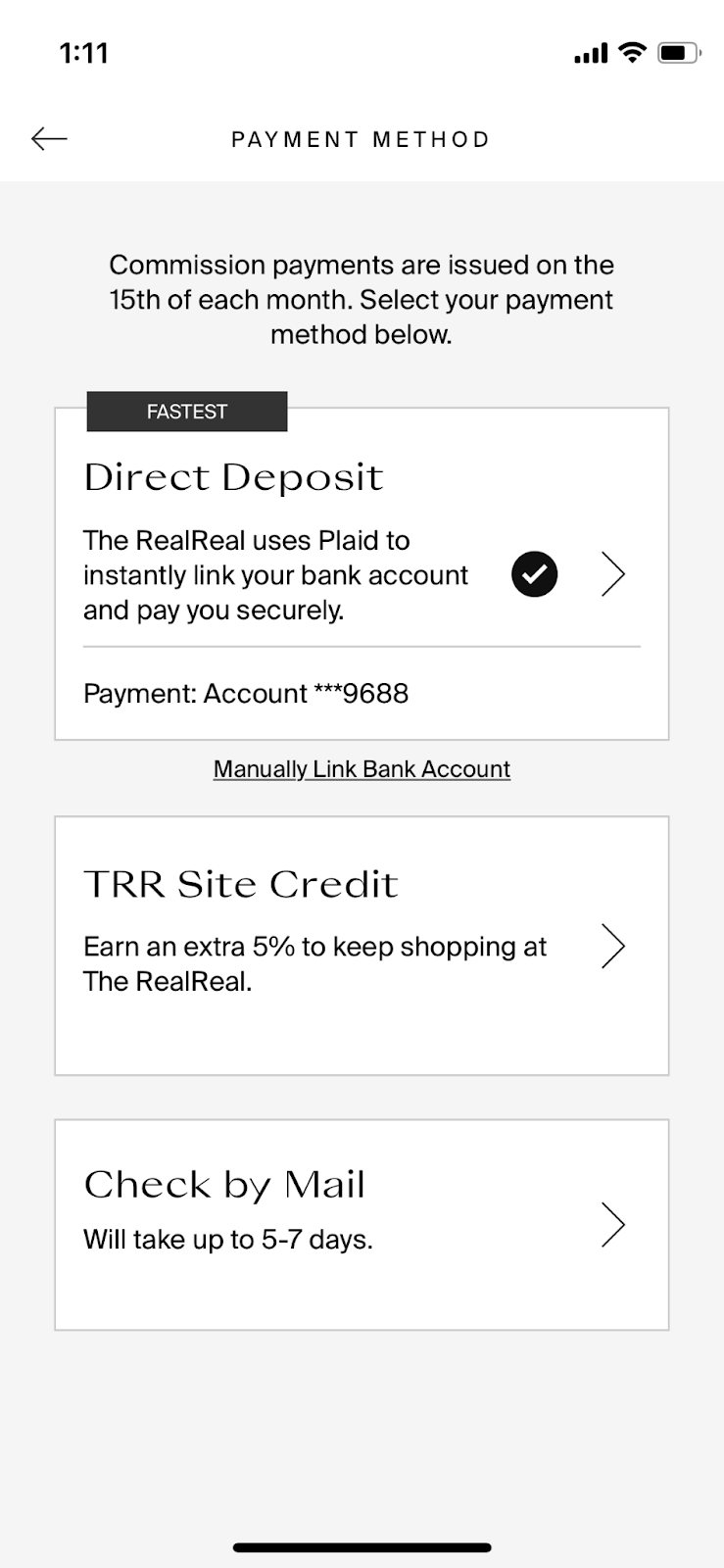This screenshot depicts a user interface for selecting a commission payment method on The RealReal website. The background of the section is light gray with three white rectangular options for payment methods, arranged vertically. 

At the top left, there's an arrow pointing to the left next to the number "111" and the phrase "payment method." Below this, a highlighted message states: "Commission payments are issued on the 15th of each month. Select your payment method below."

The first white box is for Direct Deposit. It includes some text indicating: "The RealReal uses Plaid to instantly link your bank account and pay you securely," followed by a checkmark indicating the current selection. Below, it shows the linked payment account with the masked account number "****9688," accompanied by an option to manually link a bank account.

The second white box is for earning TRR (The RealReal) site credit, which includes an enticing offer: "Earn an extra 5% to keep shopping at The RealReal."

The third white box offers the option to receive a check by mail, with an annotation that this method will take up to five to seven days.

The bottom middle of the section features a prominent black bar.

Overall, the design is clean and user-friendly, guiding users to easily select their preferred payment method.